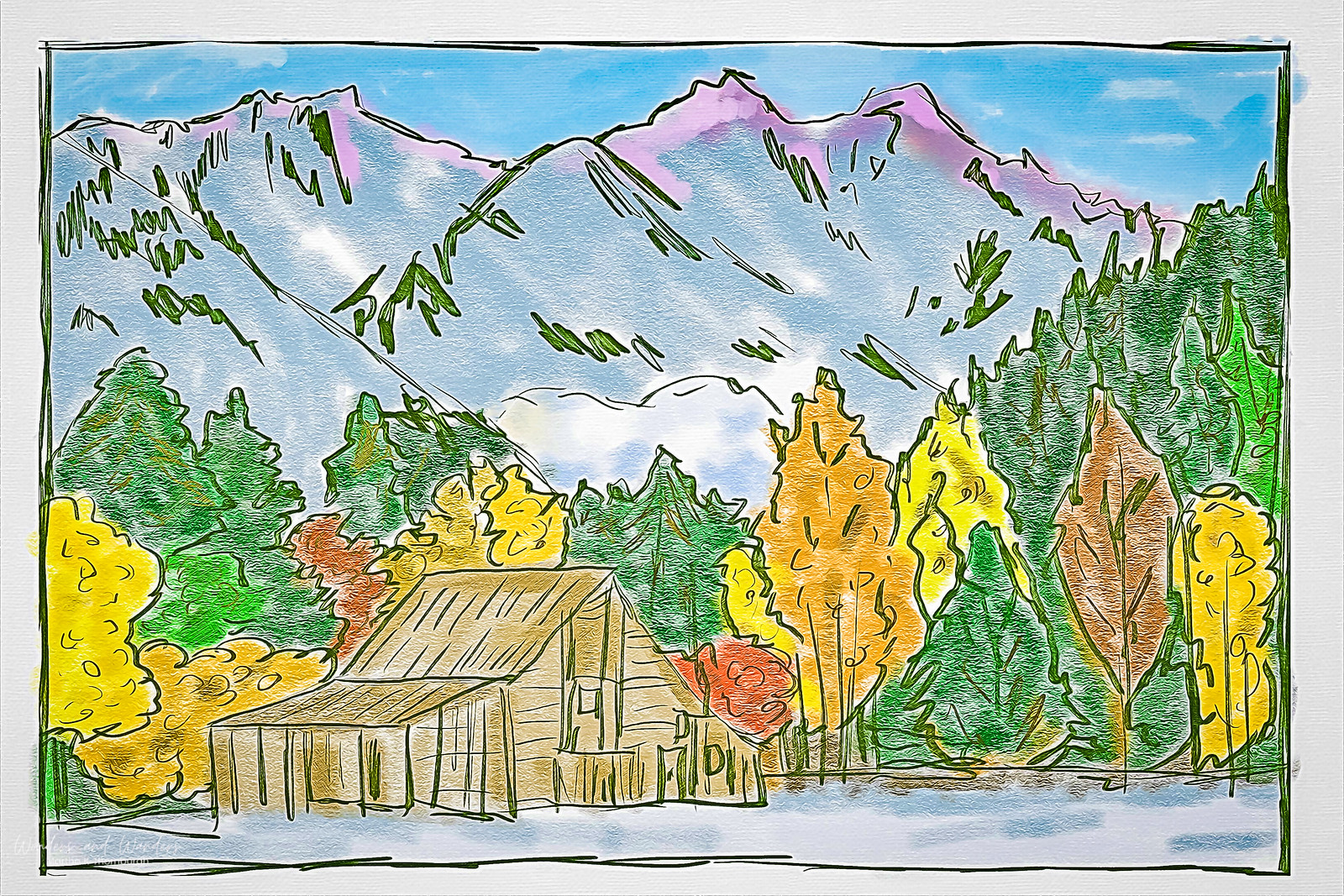This detailed image is an artistic illustration, possibly a painting or a pencil drawing, depicting a rustic wooden cabin with a prominent A-frame roof and an open-sided porch. The cabin, characterized by its unfinished brown wood exterior, is surrounded by a vibrant array of trees in various autumnal hues—green, yellow, orange, and red—indicating the changing seasons. The setting suggests it may be situated near a lake, as the ground below it is shaded blue. In the background, a majestic snow-capped mountain range extends across the width of the image, with some green patches breaking the blanket of snow and a touch of purple near the peaks. The scene is completed with a clear blue sky at the top, adding to the overall serene and picturesque quality of the artwork.